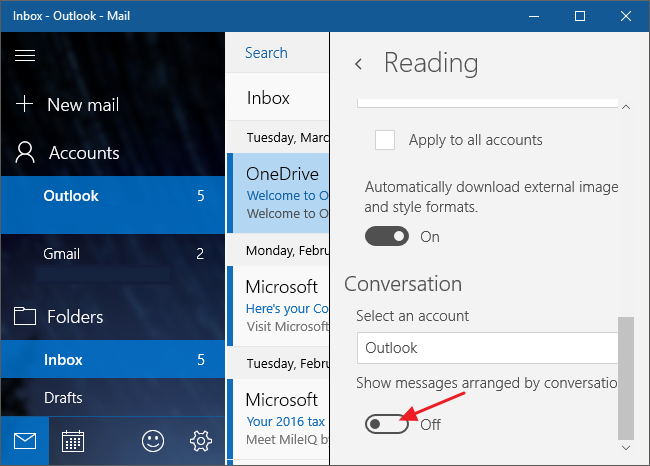In this image, we observe a screenshot of an Outlook Mail interface. At the top, within a blue header, "Inbox - Outlook Mail" is prominently displayed. Below this header, situated on a dark background that appears to be black with subtle blue highlights, several options are listed: "New Mail" followed by "Accounts," "Outlook," "Gmail," "Folders," "Inbox," and "Drafts." Along the bottom of this dark section, a row of icons is visible, including a letter icon, a calendar icon, an emoji icon, and a settings icon.

To the right, additional options are partially obscured by a pop-up box. Although the full text is cut off, readable segments include "Inbox," "OneDrive," "Microsoft," followed by another truncated "Microsoft." The obscuring pop-up box prominently displays the word "Reading," with an option "Apply to all accounts," and a toggle switch for "Automatically download external images and style formats," which is set to "On." Below this, the label "Conversation" appears, with a prompt to "Select an account," specifying "Outlook." The option "Show messages arranged by conversation" is presented with its corresponding toggle switch set to "Off."